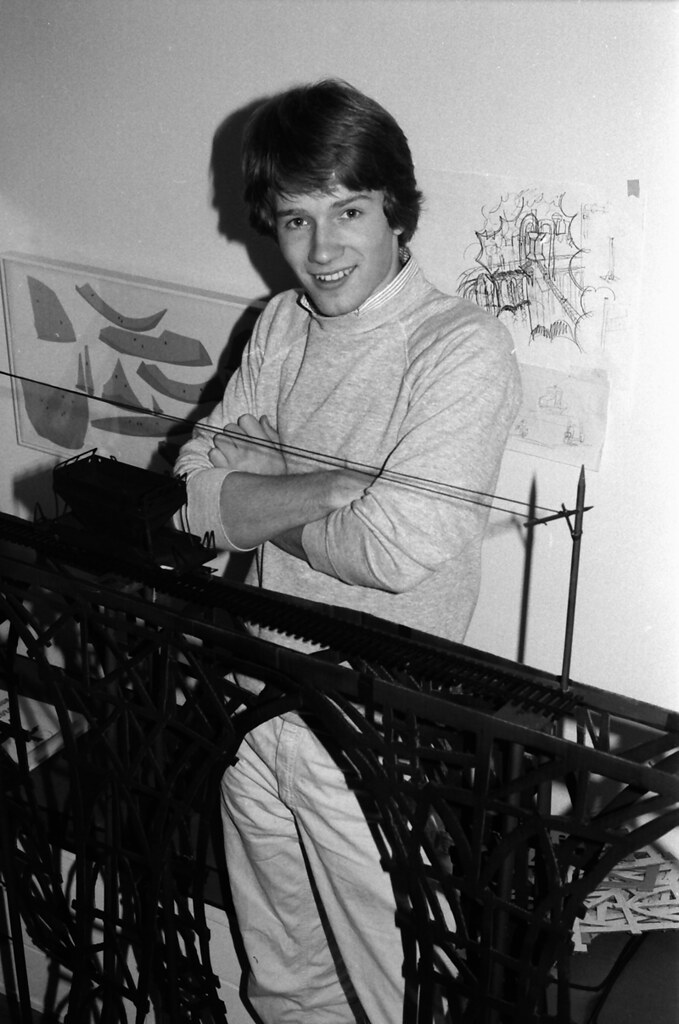In this grayscale photograph, a young man with black, swept-over hair stands in the center of the image, looking slightly towards the camera. He is dressed in a gray turtleneck sweater and white pants, with his arms crossed and an expression that appears friendly, as he shows his teeth in a subtle smile. The scene is set indoors, possibly in a museum, as suggested by the clean, organized setting.

The most prominent foreground feature is a detailed model of a bridge, complete with a train track and a miniature train on top. Accompanying the bridge model is a scale model of a power line, adding to the intricate realism depicted. Behind the man, a piece of artwork or a hand-drawn plan—possibly framed or under glass—hangs on the white wall, implying that the man might be an engineer or architect presenting one of his designs.

The only shades in the image range from pure white to deep black, creating a wide array of gray tones that emphasize the photograph’s vintage appeal. There is no visible text within the image, allowing the structured background and the detailed models to capture the viewer's attention.